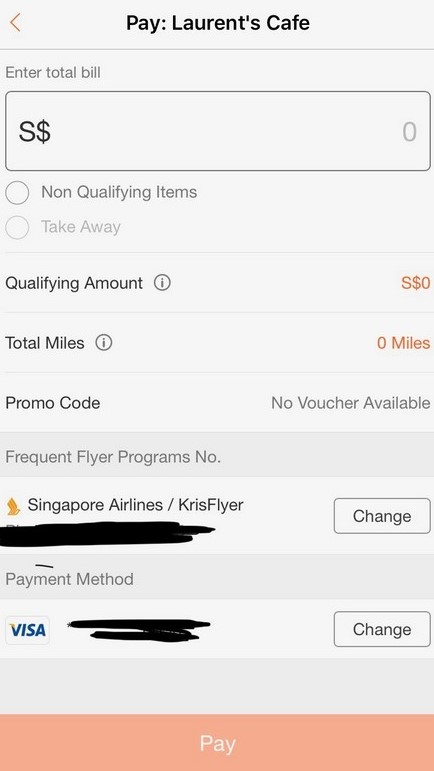The image showcases a mobile payment screen for Laurence Cafe. At the top left corner, there's a back arrow in yellow followed by the page title "Pay." Directly beneath the title, a thin light green line accentuates the section heading. The screen prompts the user to "Enter Total Bill," displaying an 'S' followed by a dollar sign and an empty field for input. A light gray zero resides on the far right within the input box, which is encased in a thin, dark to medium gray border with rounded corners.

Below the input area, there are several unchecked circular options labeled "Non-qualifying terms" and "Takeaway" in lighter text. Further down, an orange number '0' is shown next to "Qualifying Amount: S" and "Total Miles: 0 miles." Information icons are situated to the right of these text lines.

The next section reads "Promo Code" which states "No Voucher Available" to its right. Adjacent to this, a light pink bar labeled "Frequent Flyer Programs Number" appears. Underneath, on a white background, the text "Singapore Airlines / KrisFlyer" is partially obscured with a "Change" button on the right and the Singapore Airlines logo on the left. The cardholder’s info is scratched out.

The "Payment Method" section is highlighted with a light pink banner, followed by a white field displaying the Visa logo and a blacked-out card number. There is another "Change" button beneath this on a pink strip.

At the bottom of the screen, a darker pink bar features a prominently displayed white "Pay" button, indicating the final step for completing the transaction.